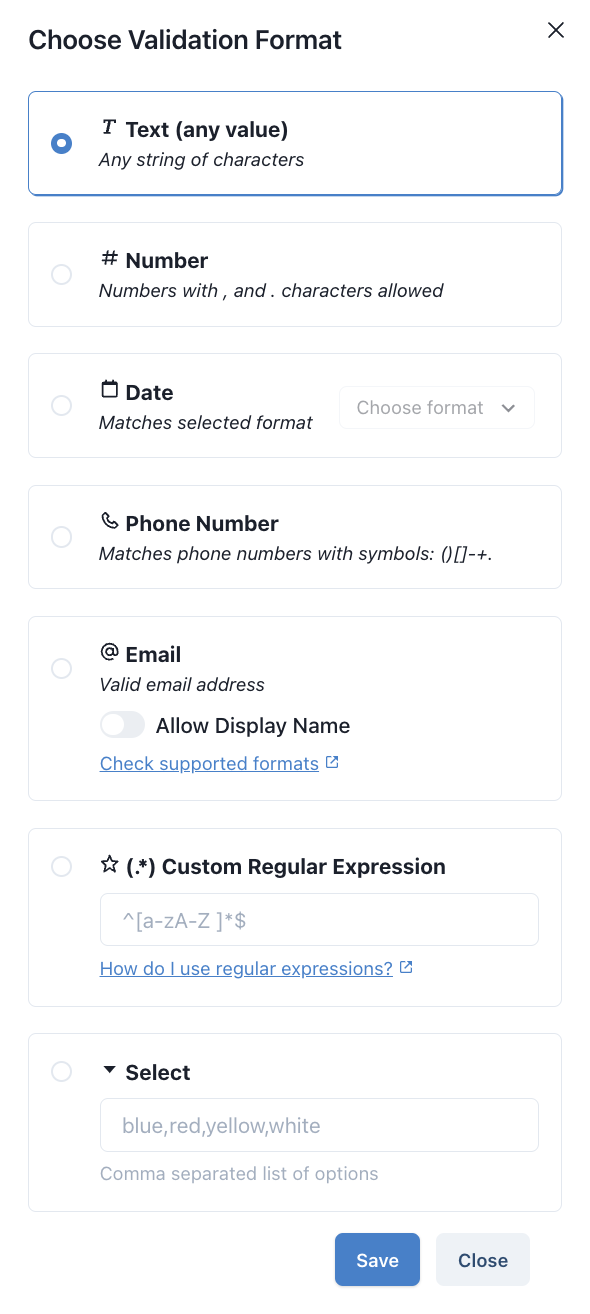This image appears to be a screenshot taken on a cell phone, depicting a user interface for selecting a validation format. At the top, it displays the title "Choose Validation Format" with an 'X' icon on the right to close the page. Below, there is a rectangular box labeled "T, Text," with the description "Any value, any string of characters." The option is selected, indicated by a blue-filled circle.

Further down, another option is labeled "# Number," allowing "Numbers with commas and periods." This is followed by a separate box showing a tiny calendar icon next to the word "Date," with an instruction to "Choose format." Under "Date," it notes "Matches selected format."

Next, there is an option for "Phone Number," accompanied by a small handset icon. It specifies "Matches phone number with symbols: parentheses, square brackets, minus, plus sign, and period."

Below is the "Email" option, noting "Valid email address" with an additional option to "Allow display name" and a note to "Check unsupported formats."

The subsequent section features a box labeled "Custom Regular Expression," containing symbols: a star, parentheses, a period, an asterisk, followed by the closed parentheses. Inside this box, it includes an upward arrow and square brackets containing "a-z" in lowercase and "A-Z" in uppercase, followed by a closed bracket, an asterisk, and a dollar sign, with a tooltip explaining "How do I use regular expressions?"

Finally, there is a section labeled "Select," with options listed as "Blue, Red, Yellow, White," in a comma-separated list. At the bottom, there is a "Save and Close" button.